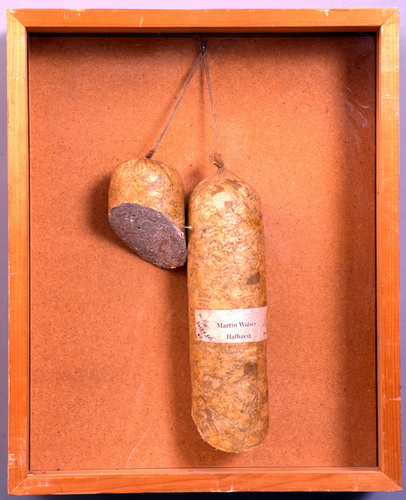This intriguing photograph captures an abstract artwork, displayed inside a shadow box, featuring two pieces of meat, resembling varieties like kielbasa, sausage, bologna, or pepperoni. The primary piece is a substantial sausage, wrapped and tied off at the ends, showcasing an evident white label on the right side reading "Martin Weber Halberd." This sausage, brown in color, hangs vertically from a piece of twine affixed to a nail at the top of the box. Adjacent to it is a sliced section, perhaps an eighth of the whole piece, also suspended by a string.

The framing of the artwork is notably rustic, constructed from wood that appears to have been painted and sanded, revealing underlying whitish areas due to scratches and marks. The background inside the frame is a terracotta red, enhancing the display's contrast. This carefully arranged composition provides a unique and detailed visual appeal, highlighting both the form and texture of the meats against the backdrop.